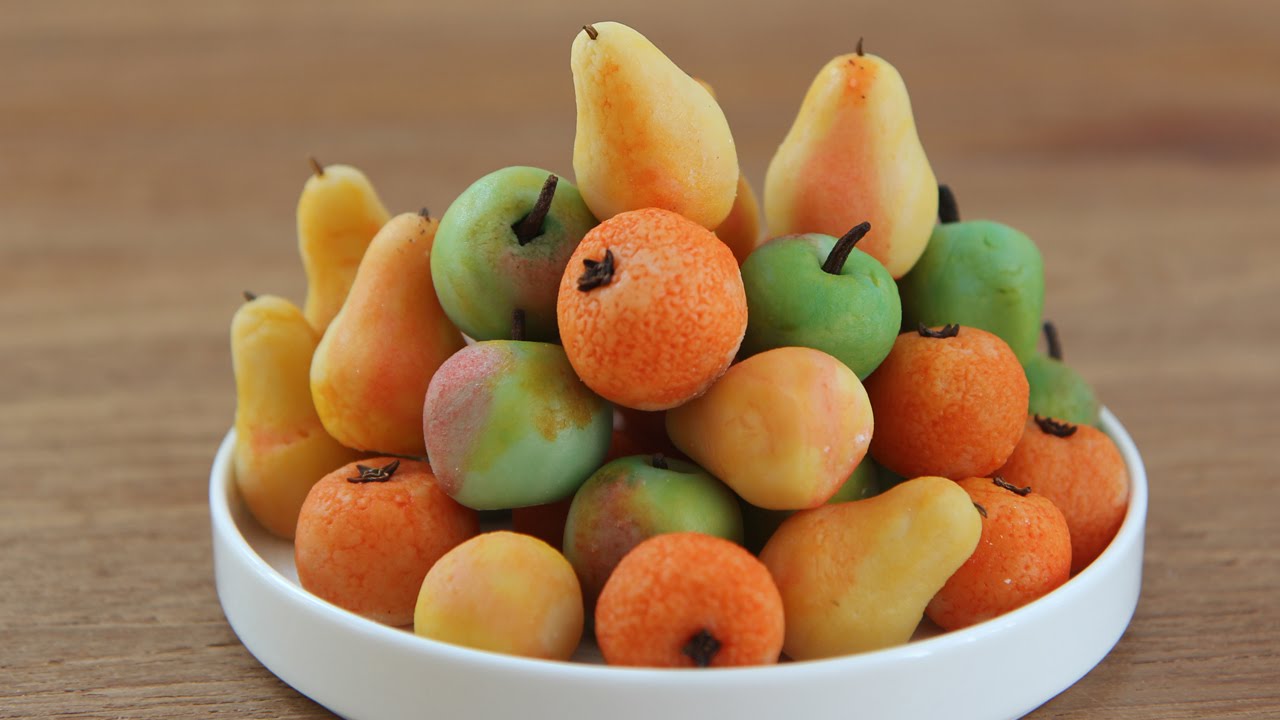In this color photograph taken in landscape orientation, the focus is on a white ceramic dish with a raised edge, elegantly placed on an unfinished medium brown wooden surface. The dish is filled with an assortment of meticulously detailed, miniature fruits, resembling those possibly crafted for a dollhouse. Among the fruits are textured oranges, each with a small brown stem, realistic green apples some of which feature red streaks with pointy dark brown stems, and yellow pears highlighted with touches of red and tiny brown stems. There is also an unidentifiable round yellow fruit added to the mix. The photograph's depth of field causes the background to blur slightly, emphasizing the intricate realism of the miniature fruits which appear to be made from a material akin to modeling clay.